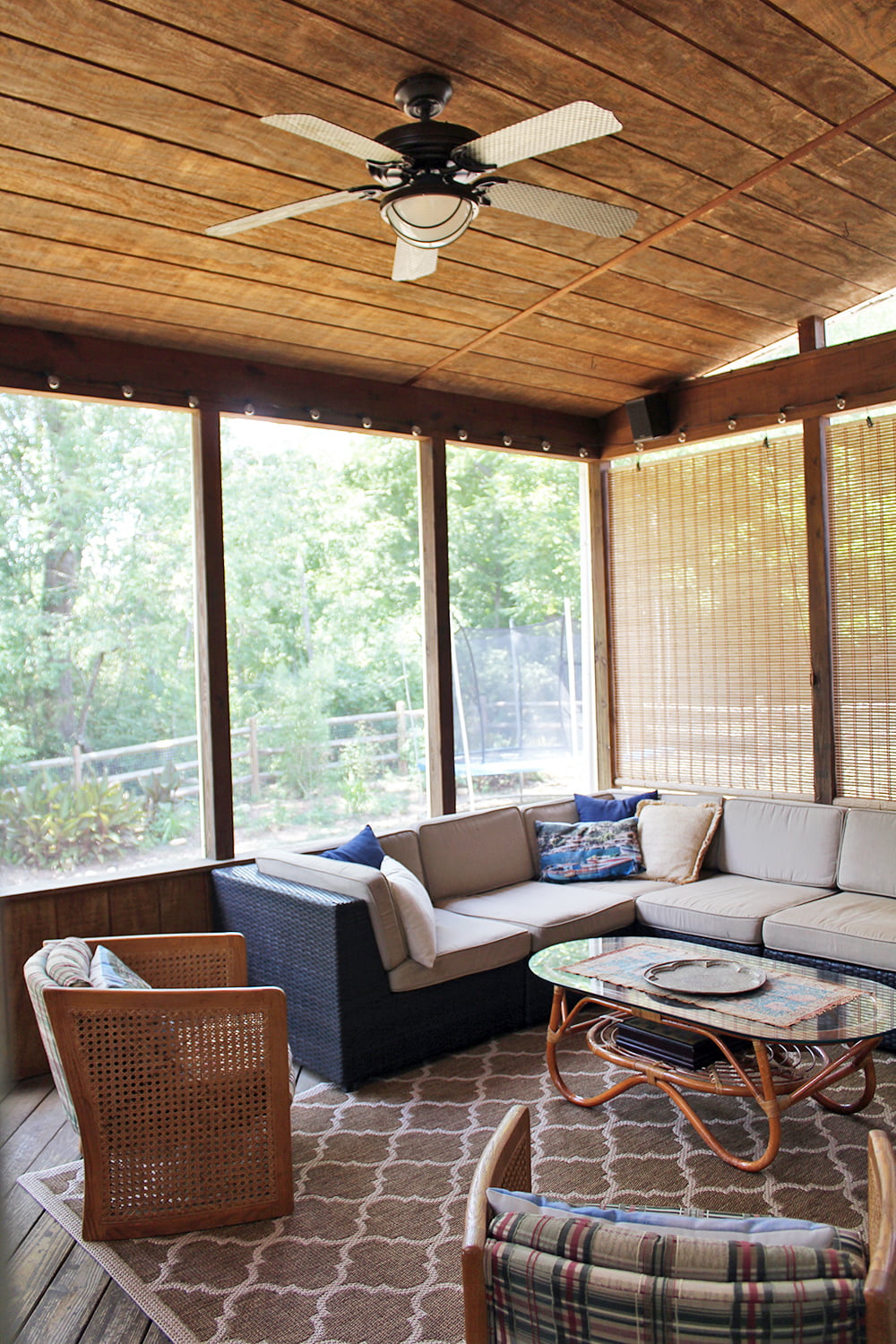This is a photograph of a stylish living room that exudes a minimalist yet warm design. The room is enveloped almost entirely by large, floor-to-ceiling windows, offering an unobstructed view of the surrounding forested area. Outside, a wooden fence borders the property, and a trail can be seen winding its way into the dense greenery.

Inside, the room features a slightly sloped wooden ceiling with a fancy ceiling fan complete with a dome light. Wooden frames border the windows, enhancing the natural aesthetic. The highlight of the room is a spacious corner sectional sofa, upholstered in gray fabric with blue accents at the base and adorned with several pillows.

Complementing the sofa, there are two wicker-style chairs with soft cushioning and wooden sides. A brown rug with hints of white anchors the furniture, resting above a polished wooden floor. A central coffee table, featuring wooden wicker-like legs and a glass top, holds an empty silver pan, adding a touch of elegance.

The overall ambiance is clean and sophisticated, reminiscent of a feature in Architectural Digest, emphasizing both natural light and wooden elements to create a welcoming and serene atmosphere.